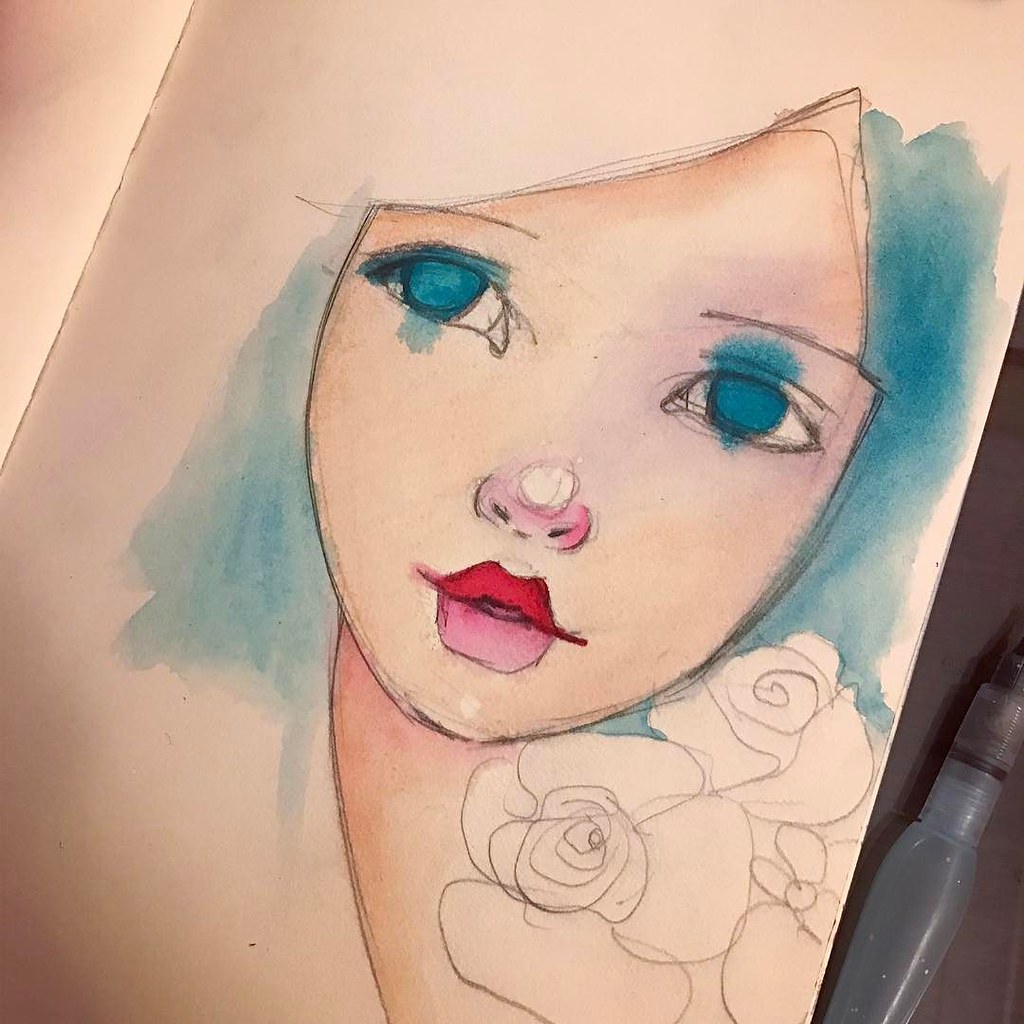This image captures a photograph of an unfinished piece of artwork, likely created using a combination of pencil drawing and watercolor paint, on a beige-pink background. The central focus is a young woman's face, which occupies the majority of the tilted canvas. Her face, outlined with incomplete, dark pencil lines, features strikingly bold, blue-green eyes with watercolor extending above and below them. The eyes, devoid of irises, contribute to a dreamy, neutral expression. She has prominent red lips and a small pink nose with a white highlight on its tip.

The hair framing her face is partially colored in the same blue-green hue as her eyes, covering areas along the sides of her head but leaving the top unfinished. Her eyebrows are lightly penciled in with slight slants. Her neck extends awkwardly to one side, drawn with a faint indication of flesh tone. Adjacent to her neck, in the lower right corner, are pencil sketches of roses that have yet to be colored.

The entire artwork is slightly askew to the right within the photograph. In the bottom right corner of the image, outside the artwork, there is an empty paint bottle, hinting at the ongoing nature of the piece. Both the composition and the incomplete state of the artwork evoke a sense of work-in-progress.